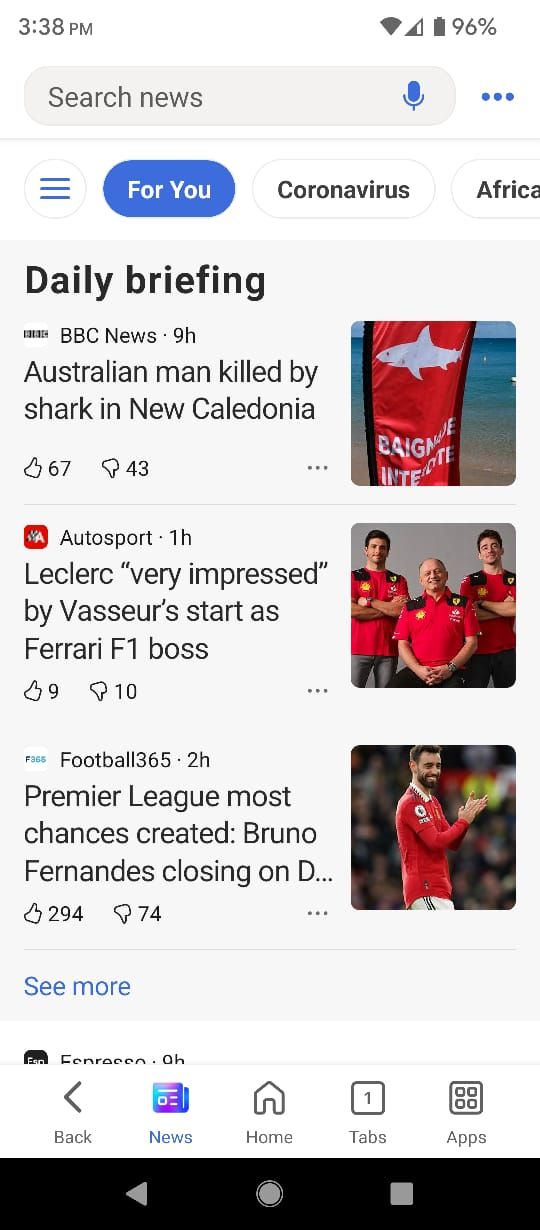This is a screenshot of a news app on a mobile device, showcasing its user interface and various functionalities. At the top of the app, a search bar is prominently displayed, featuring the text "Search news." To the right of the search bar is a blue microphone icon, allowing users to perform voice searches. Adjacent to this, on the far right, are three vertical blue dots, typically indicating access to the app's settings menu.

Below this top navigation area, there is an icon resembling a circle with three horizontal blue lines, often used to tailor or customize news feeds based on specific interests. Following this, there are three prominent category links labeled "4U," "Coronavirus," and "Africa," allowing users to quickly access news related to their preferences, updates on the coronavirus pandemic, or news specific to the African continent.

The main content area below these links features a daily briefing with several listed articles. The highlighted articles include headlines such as "Australian man killed by shark in New Caledonia," "Leclerc very impressed by Vasseur's start as Ferrari F1 boss," and "Premier League most chances created, Bruno Fernandes closing." There is a "See More" link provided for users to access additional news articles.

At the bottom of the screen, a navigation bar is present with icons for "Back," "News," "Home," "Tabs," and "Apps," helping users to easily navigate through different sections of the app.